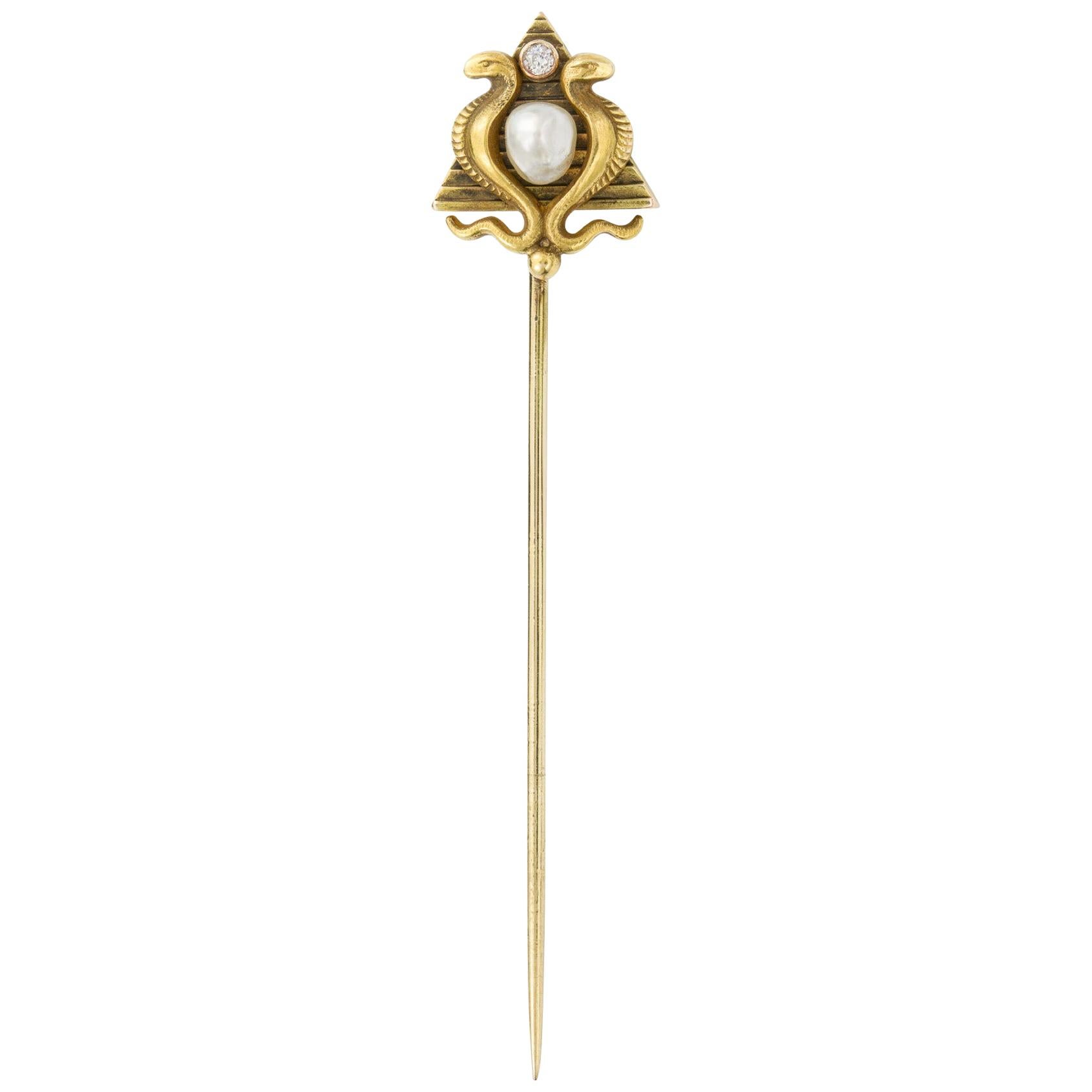This image showcases a highly ornate, antique accessory against a plain white background, making it the sole focus. The item, initially resembling a hairpin or hat pin, is a diamond pin with a gold and silver aesthetic. The pin features a slender, golden body extending into a long needle, suggesting its use in securing hair or as a decorative hat accessory. The highlight of the pin is its intricately designed triangular top. Within this gold triangular frame are two gold-colored snakes winding up from the base to the apex, their heads facing opposite directions at the top. The center of the triangle hosts a circular area, which houses what appears to be a small, embedded diamond or pearl, adding to the pin’s opulent appearance. The absence of any text, numbers, or any discernible background elements emphasizes its likely antique origin and singular beauty. Estimations suggest the pin measures around three to four inches in length, though the exact size remains unclear due to the lack of reference points in the image.